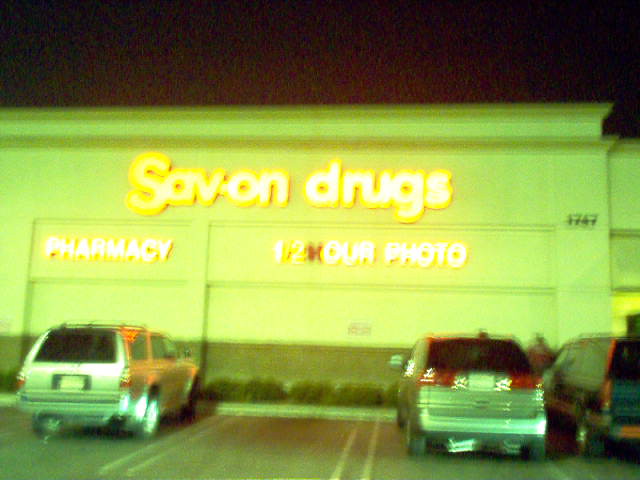This is a nighttime photograph of a large, single-story pharmacy with a high ceiling, situated at 1747, as indicated by the number on one of the building's columns. The building exterior is light green with a brown brick base. The prominent store signage includes "Save On Drugs" in big white letters outlined in yellow, which have a neon-like glow. Below it, "Pharmacy" and "1 Hour Photo" are also displayed in white trimmed with yellow. The image, though somewhat blurred, shows cars parked in front of the store. A silver SUV is on the left, while to the right are another silver SUV and a turquoise-colored truck. A curb with green bushes and dividing lines in the parking lot is visible. The black night sky contrasts with the illuminated storefront, contributing to the vivid nocturnal ambiance. A person stands near one of the cars, adding a subtle human element to the scene.